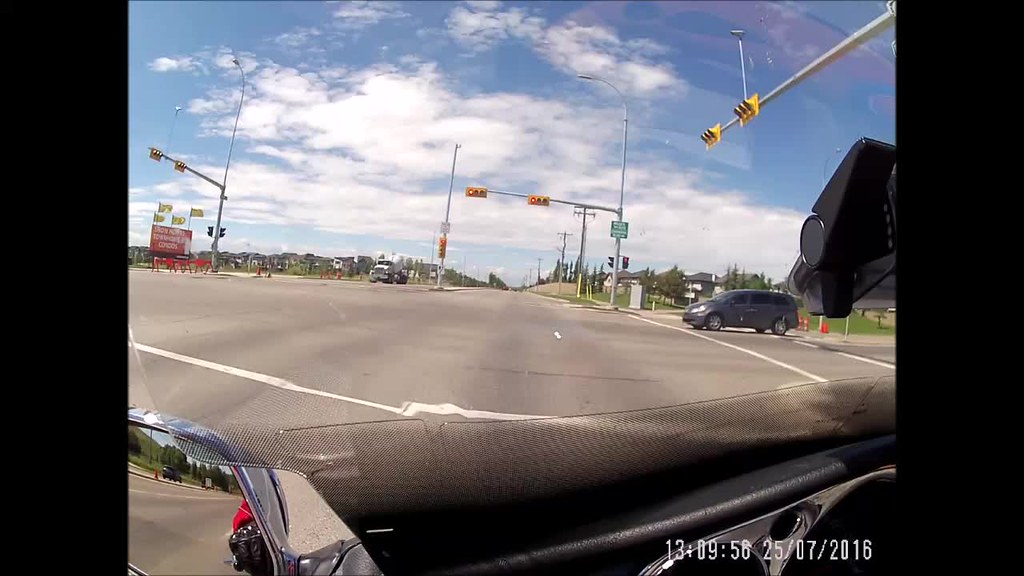The photograph, taken from inside a car, captures part of the vehicle's black dashboard with chrome accents, along with the rearview mirror positioned in the lower left corner. The car is stopped at an intersection on a highway that has at least two lanes in each direction. Visible ahead are two red stoplights hanging above the intersection. In the distance, a dark grey minivan is seen waiting in the pedestrian crosswalk on the cross street to the right. Behind the photographer's vehicle, a hint of something red is visible. To the left, slightly above the midpoint of the frame, a red sign stands, although its content is unclear. The landscape appears flat with sparse surroundings, indicating the photograph was taken in an area with substantial highways.